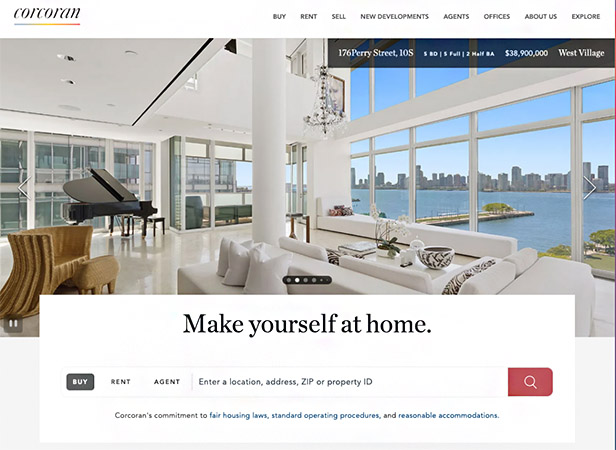The website titled "Coro Corcoran" features a sleek design with a black-on-white color scheme. At the top, there's a navigation bar with several options: Buy, Rent, Sell, New Developments, Agents, Offices, About Us, and Explore.

Just below the navigation bar, there is a photo of a pristine, all-white living room. Everything in the room—the furniture, walls, floor, and ceiling—is white, creating a seamless and sophisticated look. The only contrasting elements are a brown chair and a black piano, adding a touch of warmth and elegance. Beneath the image, the text "Make Yourself at Home" is prominently displayed.

Further down, there is a search bar with options to buy, rent, or find an agent. Users can input a location, address, zip code, or property type and click a distinctive red search button. Additional text affirms "Coro Coren's commitment to fair housing laws, standard operating procedures, and reasonable accommodations."

On the right side of the photograph, overlaid on a black band, is detailed property information: "176 Perry Street, 10S. 3 bedrooms, 3 full, 2 half baths. $39,900,000. West Village." The property is described with a stunning view of a harbor and a cityscape in the distance, adding to its luxurious appeal.